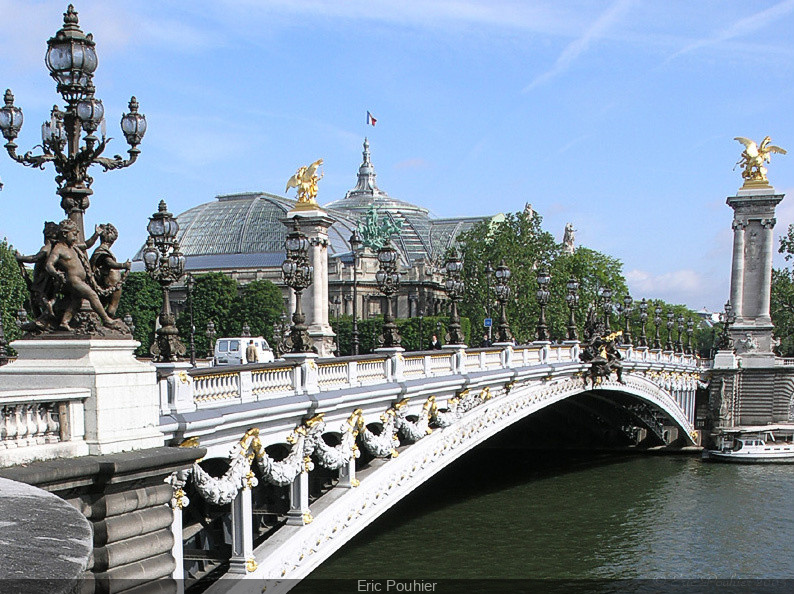The photograph captures the ornate and historical architecture of the Seine River in France. Dominating the scene is a majestic white bridge with gold accents, featuring a distinct arch shape. The bridge is adorned with elaborate plaster embellishments depicting human faces, flowers, and leaves. Atop its pillars are iron sculptures of cherubs, possibly holding grapes, which add to the bridge's intricate design. The most striking elements are the two golden, winged statues with figures riding them, perched on high plinths at either side of the bridge. In the foreground, slightly to the left, a stone statue of children encircling a light fixture can be seen. Below the bridge, the river's greenish waters flow, with a white boat visible on the side. A bus and a small white van are captured driving over the bridge, adding a touch of contemporary life to the historic setting. In the background, a significant building with a blue, white, and red French flag atop it can be seen, reminiscent of a Versailles-like palace with a glass roof. The bottom of the image bears the name "Eric Polyer" in white letters.